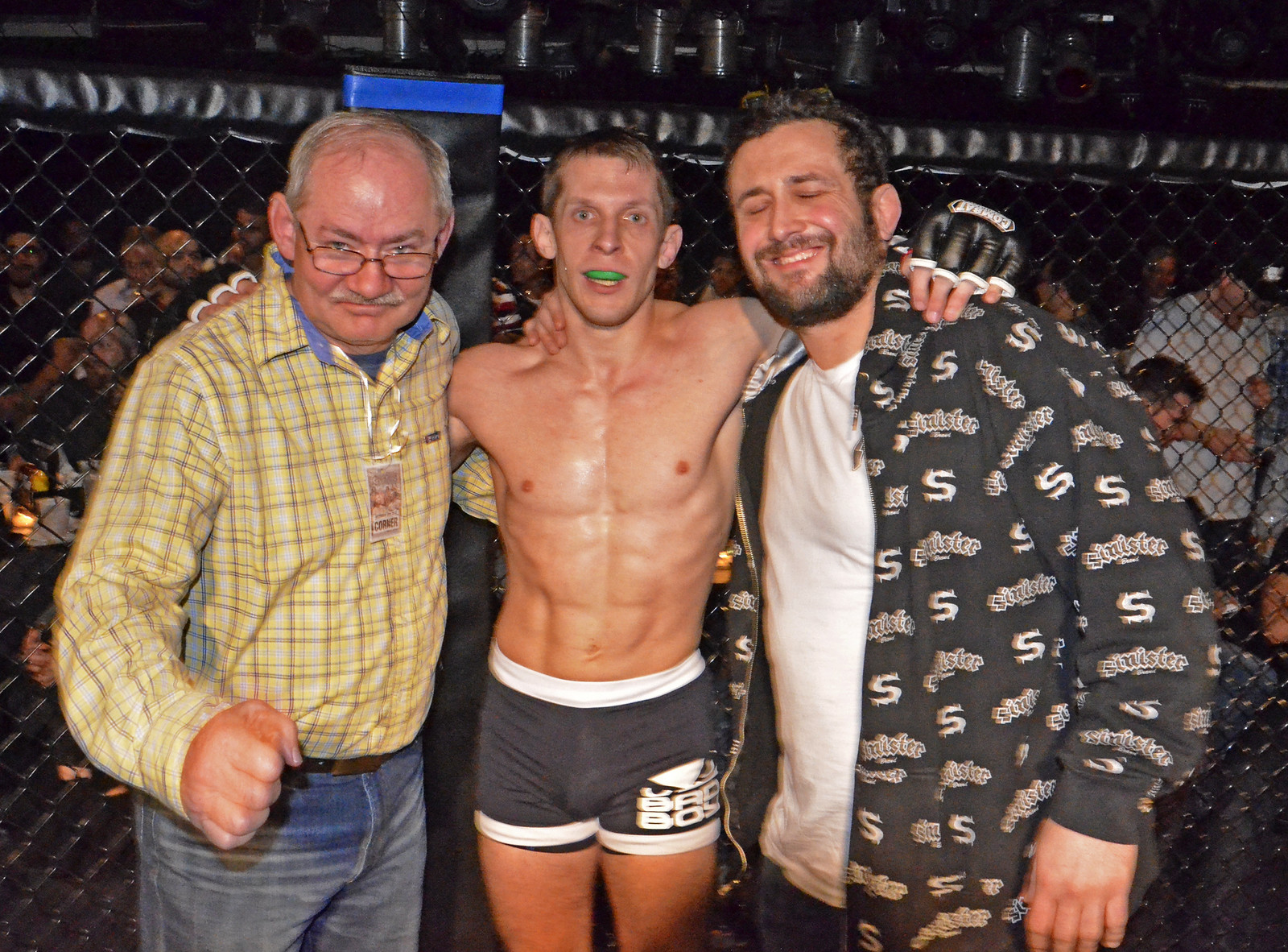In this wide rectangular photograph, taken at a mixed martial arts event, three men are posing inside a boxing ring surrounded by a black-gated, chain-link cage with a padded black border. The man in the center is a physically fit, shirtless fighter with light skin, short blond hair, and a green mouth guard. He is wearing black spandex shorts with white borders and white "Bad Boy" lettering accompanied by a cartoon-eye logo. His muscular arms are wrapped around the two men on either side of him. 

On the left stands an older man with white hair and a mustache, donning a long-sleeved yellowish-brown plaid shirt tucked into blue jeans, fastened with a belt featuring a gold buckle. He sports black-framed reading glasses and a lanyard with a tag. One of his fists is raised in a celebratory gesture while his other arm wraps around the fighter. 

To the right, a younger man with a curly brown hair and a short beard is smiling with closed eyes. He is dressed in a gray shirt topped with a black jacket featuring a white design resembling a dollar sign. His blue jeans complete the outfit. His arm, too, is wrapped affectionately around the fighter. 

Behind them, the cage’s black padding runs horizontally, framing the scene. A shadowy crowd of spectators peeks through the gaps in the cage, adding to the lively atmosphere of the event.